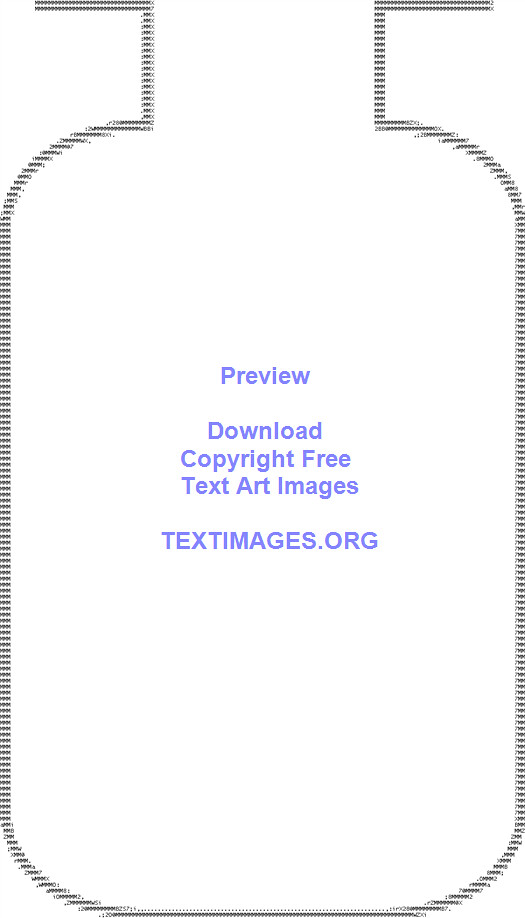This photograph features a black-and-white computerized advertisement, utilizing text art to create the image of an open bottle or cup against a plain white background. The design, crafted from text, numbers, and symbols, forms a recognizable shape reminiscent of ASCII art. Centrally positioned within the text art are five rows of pastel purple text, each word capitalized appropriately. The first row reads "Preview," the second "Download," the third "Copyright Free," the fourth "Text Art Images," and the fifth "textimages.org." The entire composition is neatly centered, making the advertisement clear and visually structured.